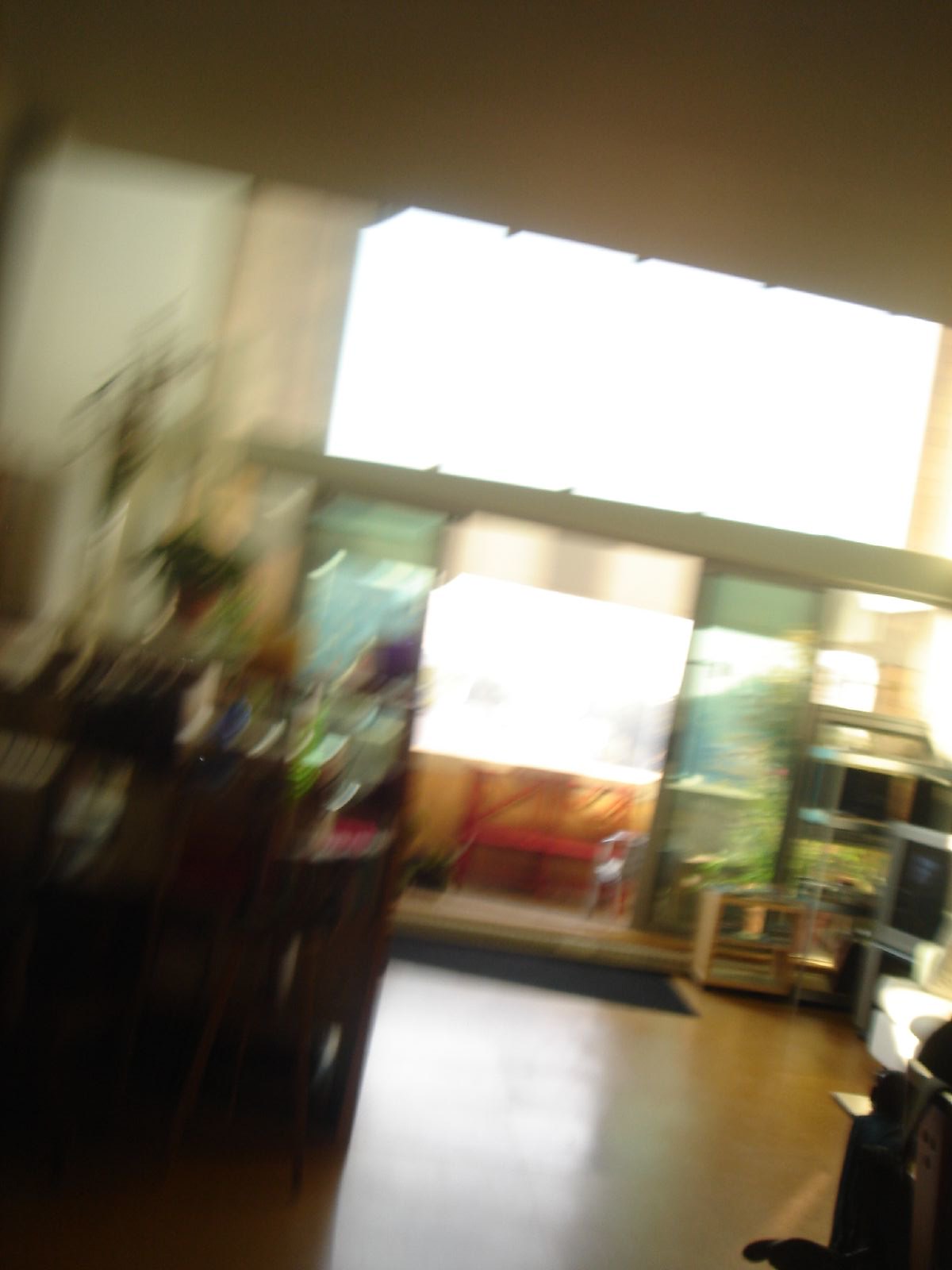This blurry photograph captures the interior of what seems to be a spacious lobby, likely situated indoors. Despite the lack of fine detail, one can discern prominent features such as a series of large glass doors or windows lining one end of the room, allowing light to spill into the space. These are accentuated by rectangular panels of bright, glowing light. Beneath one of these windows rests a distinct red bench, adding a splash of color to the otherwise muted scene. As you enter the space, a tall wooden counter, possibly serving as a check-in desk, comes into view. The presence of potted plants, albeit blurred, adds a touch of greenery and enhances the welcoming atmosphere.